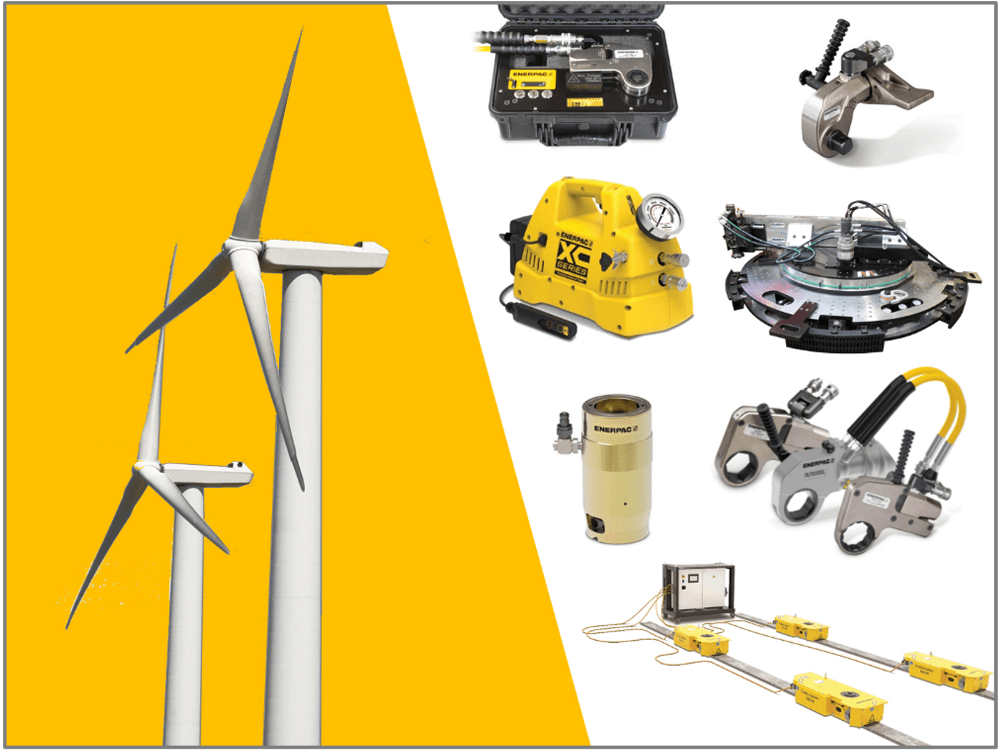The image is divided diagonally into two halves. The left half features two white wind turbines against a bright yellow background, illustrating modern power-generating machines commonly found on wind farms. The right half showcases an assortment of hand tools and mechanical devices meticulously placed over a stark white background. Positioned in rows, the top section includes a toolbox and a crane-like tool. The middle row features a flashlight and a yellow machine, likely a compressor or generator, while the lower row displays clamps, a cylindrical saw chain, and other maintenance equipment. These tools, rendered in shades of black, gray, silver, and yellow, are likely used for the upkeep and operation of the wind turbines. The image merges real equipment with a digitally crafted backdrop, emphasizing both the machinery and the tools essential for their maintenance.